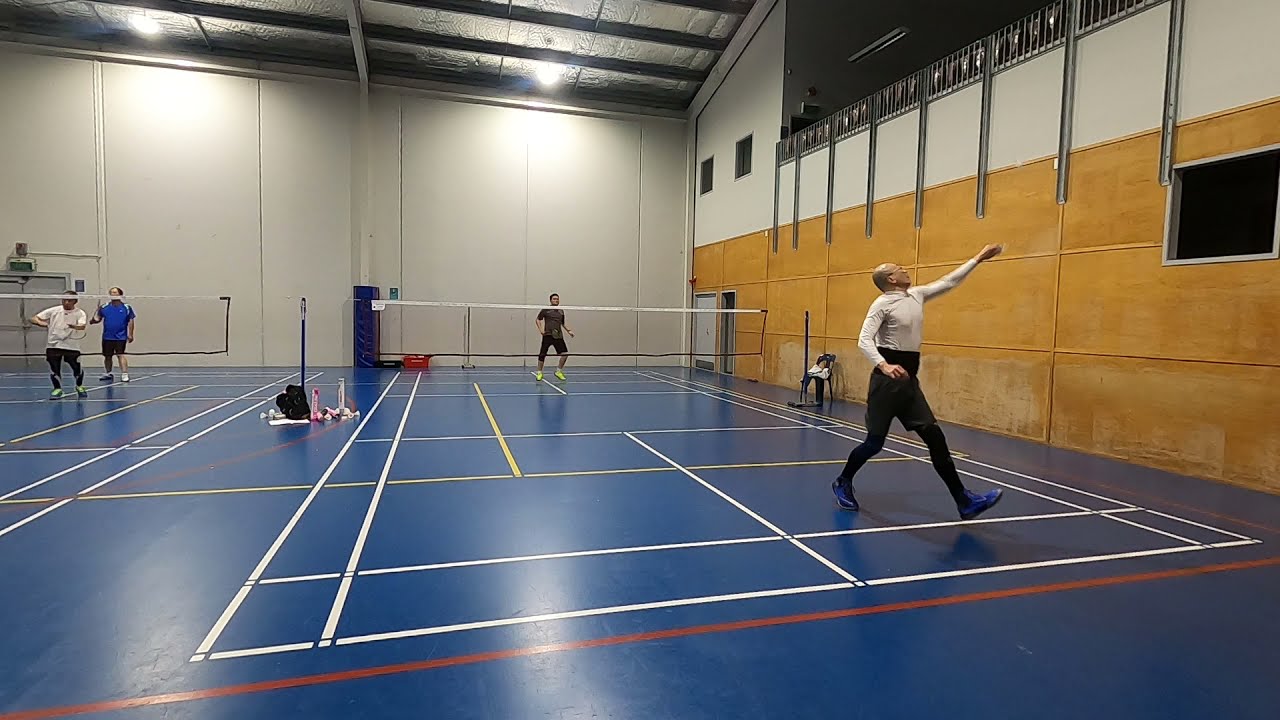In the image, a spacious indoor sports facility is depicted, featuring multiple courts that resemble tennis or pickleball courts. Each court is marked with a variety of colored lines – red, white, and yellow – painted across the blue floor, likely signifying different play areas or rules. On the primary court, there are two individuals positioned on opposite sides, suggesting a game setup. Nearby, on an adjacent court, two more people can be observed, both standing on the same side, implying that their opponents are out of the frame. The background includes a wall painted in beige and yellow, adorned with three windows, which allows natural light to filter into the brightly illuminated space, enhancing its vibrant atmosphere.